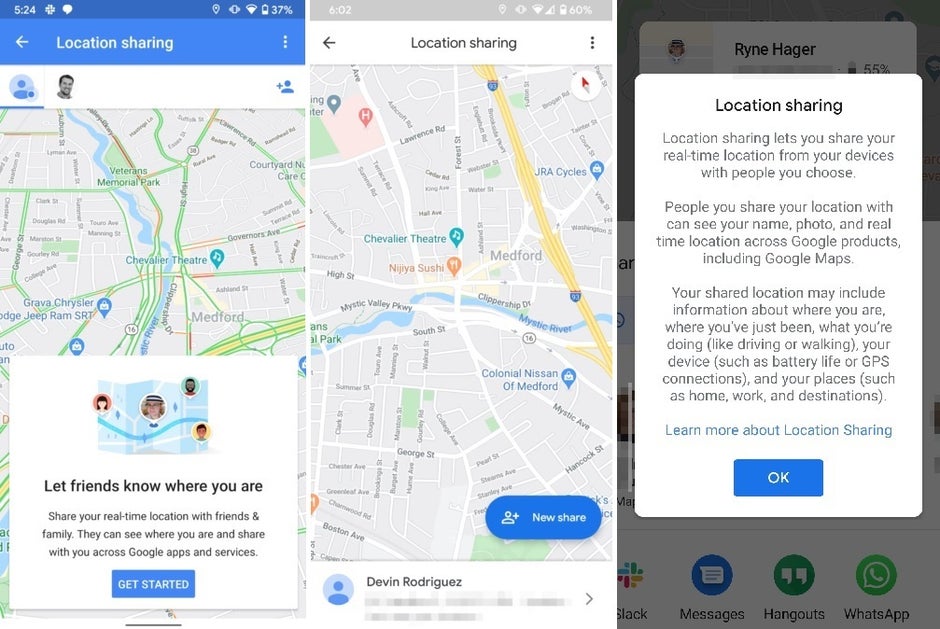This series of screenshots showcases the process of using Google’s location sharing service across various stages.

1. The first screenshot features the introductory screen of Google Location Sharing. At the center, a map is displayed with a prompt that reads, “Let friends know where you are. Share your real-time location with friends and family.” Additional text clarifies: “They can see where you are and share with you across Google apps and services.” At the bottom, a blue “Get Started” button is prominently positioned, inviting users to initiate the location sharing process.

2. The second screenshot moves further into the setup process. It also displays a map, but this time with additional control options. A significant feature is the “New Share” button, enabling users to initiate a new location-sharing session. The name “Devin Rodriguez” appears at the bottom, indicating the contact with whom the location can be shared. 

3. The final screenshot delves into the details of location sharing. It reiterates the purpose of the feature with a message that reads, “Location sharing lets you share your real-time location from your devices with people you choose.” It explains that those you share your location with will be able to see your name, photo, and real-time location across Google products, including Google Maps. Detailed informational text follows, explaining the kind of data that may be shared, such as your current activity (e.g., driving or walking), device information (e.g., battery life or GPS connection), and frequent places (e.g., home or work). The screen provides two clickable options: “Learn More About Location Sharing,” linking to further details, and an “OK” button to proceed.

This visually instructive series outlines how to enable and customize Google’s location sharing feature, crucial for users seeking to stay connected with friends and family. The layout and design are tailored to Google’s Android interface, with a noted visual difference from the iPhone version of the service.